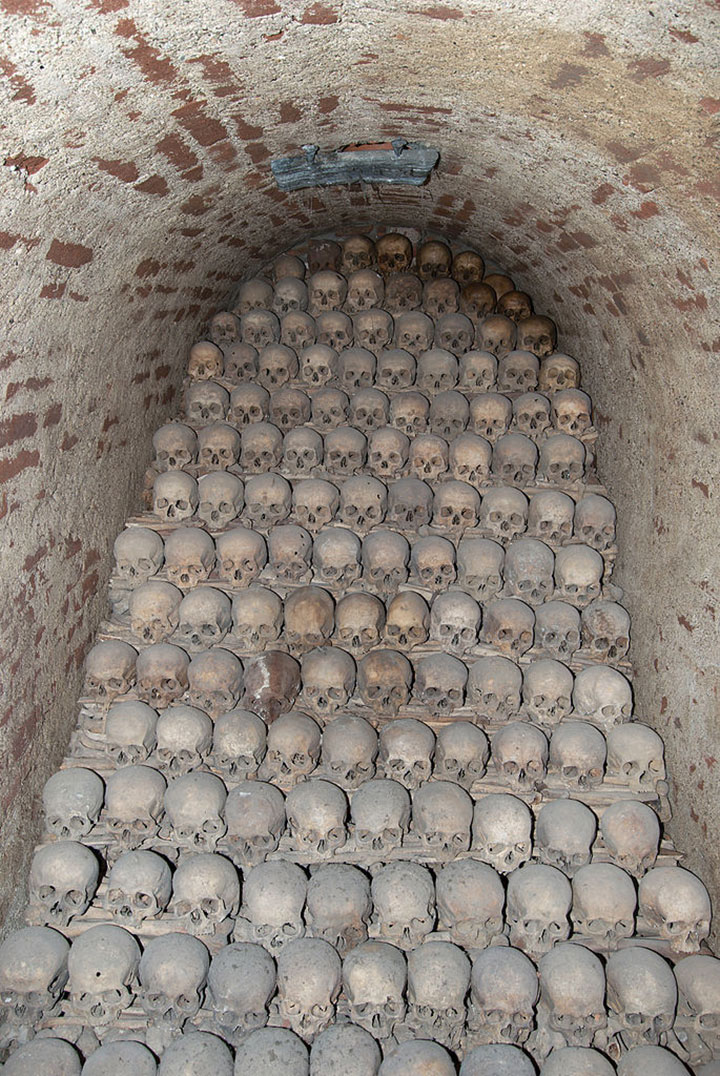The image depicts a hauntingly detailed view of a historic catacomb, likely located in Europe or Mexico. The setting reveals an arched stone chamber, resembling a man-made cave or tomb, with its walls and ceiling formed of brick colored in varying shades of brown and beige. Dominating the interior, an elaborate arrangement of countless human skulls is meticulously positioned in a stepped, staircase-like pattern from the floor to the curved ceiling of the vault. Each skull, devoid of its lower mandible, is uniformly oriented forward, presenting a solemn, repetitive visual. The skulls, appearing old and possibly charred, span approximately 10 across per row, stacking up to around 20 rows in total. The colors within the image range from gray, brown, beige, to ashy white, contributing to the eerie, somber atmosphere of this solemn, ceremonial chamber.